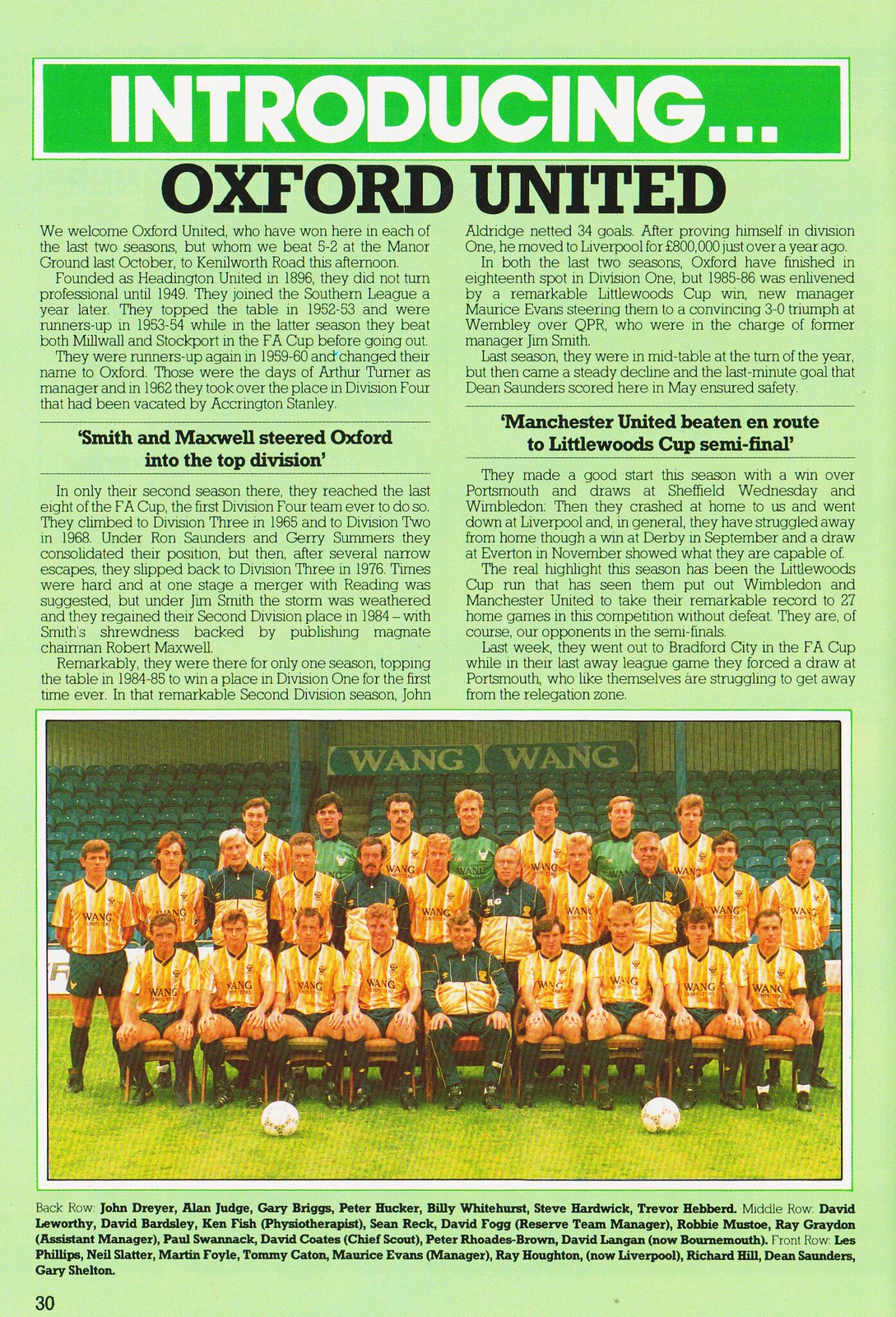This vertical rectangular image appears to be a page from a magazine or a newspaper article, rather than a poster, given the extensive amount of text. The background is predominantly lime green, and at the top, there is a darker green box with large white block letters that read "Introducing...". Just below this, in black block text, it says "Oxford United".

The main feature of the page is a two-column article about the Oxford United soccer team. In the middle of the article is a photograph of the team posing at their stadium. The players are wearing yellow jerseys paired with either black or green shorts. There are three rows of individuals: the back row consists of players standing, the middle row also standing, and the front row sitting in chairs. The coaches, distinguishable by their green and yellow jackets, are interspersed among the players. Additionally, there are two soccer balls positioned on the ground in front of the group.

In the text surrounding the photo, key highlights include the phrases "Smith and Maxwell steered Oxford into the top division" on the left and "Manchester United beaten en route to Littlewoods Cup semifinal" on the right. Below the photograph, the article lists the names and positions of all the individuals in the photo, categorized by their row: back row, middle row, and front row. The detailed layout and information suggest this is indeed a comprehensive feature article on Oxford United with a celebratory introduction.